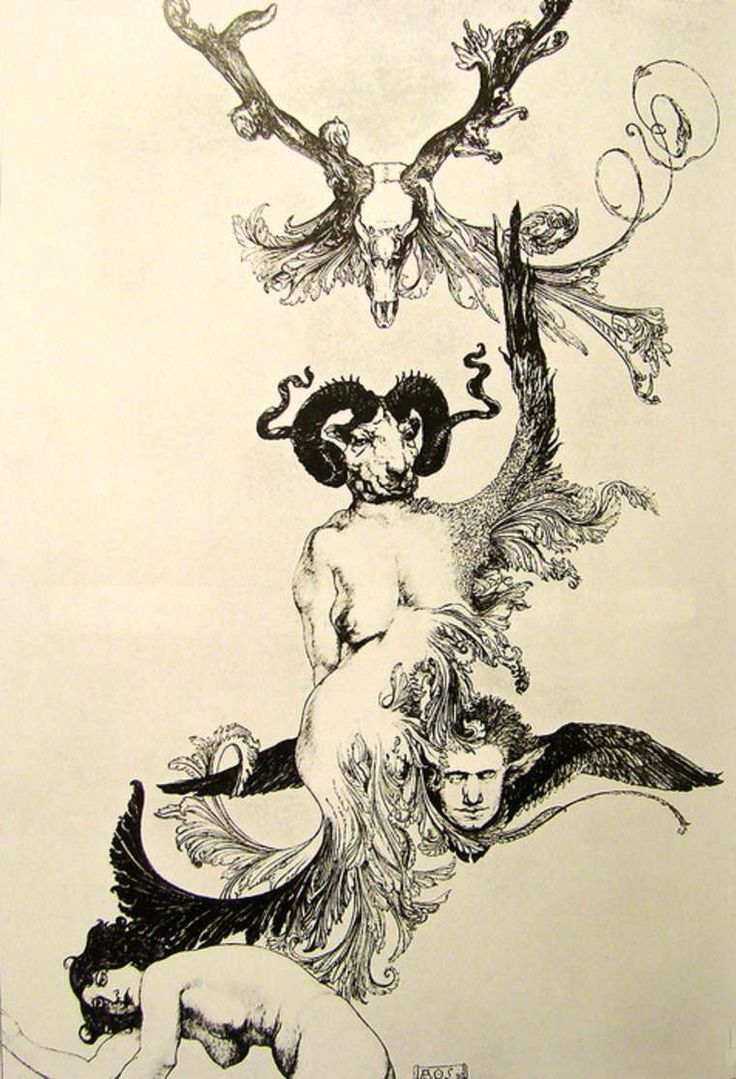This pen and ink sketch on white paper forms a complex, tree-like structure with multiple interwoven characters and abstract elements. Dominating the center is a winged male figure in flight, with feathery wings and a ram with distinctive thick black horns seated upon his back. Below him, a naked woman with dark, curly hair arches her body towards the bottom left, her breasts hanging down. The ram-like character also exhibits a human-like body, blurring the lines between human and animal. Adding to the intricate scene, a bird-like creature with a long beak and outstretched wings rises above, its feathers extending to the upper right of the illustration. To the lower right, a smaller, elf-like head with spiky hair and ears jutting out, adorned with wings on its sides, adds to the surreal composition. At the top, a detailed deer skull with antlers resembling tree limbs completes the composition, tying together the various fantastical elements into a unified, mystical tableau.